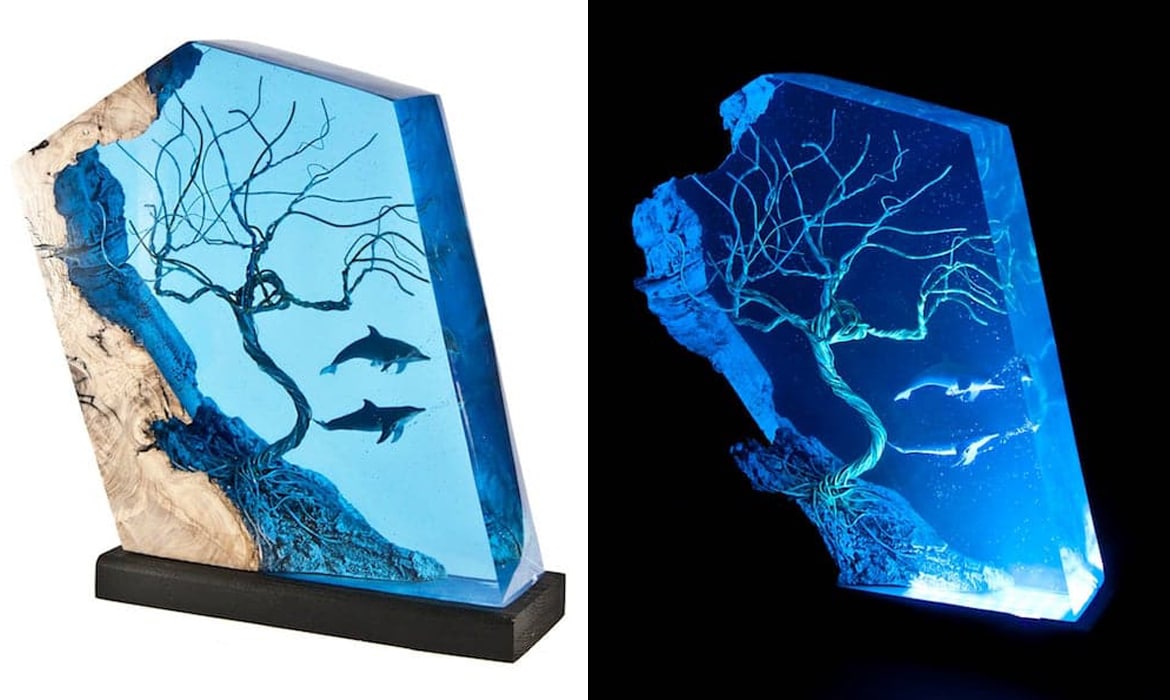This image shows two side-by-side photographs of a unique resin mold artwork piece that serves as a bookend. The piece is shaped like a slanted pentagon or diamond, featuring natural wood on the left side and clear, blue-tinted resin on the right. Inside the blue resin, a metallic tree stands, accompanied by two swimming dolphins, with air bubbles emanating from them, creating an underwater scene. The artwork sits on a black base, likely wooden. In the left photograph, the piece is placed on a black table, while in the right photograph, the scene is depicted in darkness, highlighting the illumination from within the base, which lights up the blue resin portion, making the rest of the piece blend into the black background.